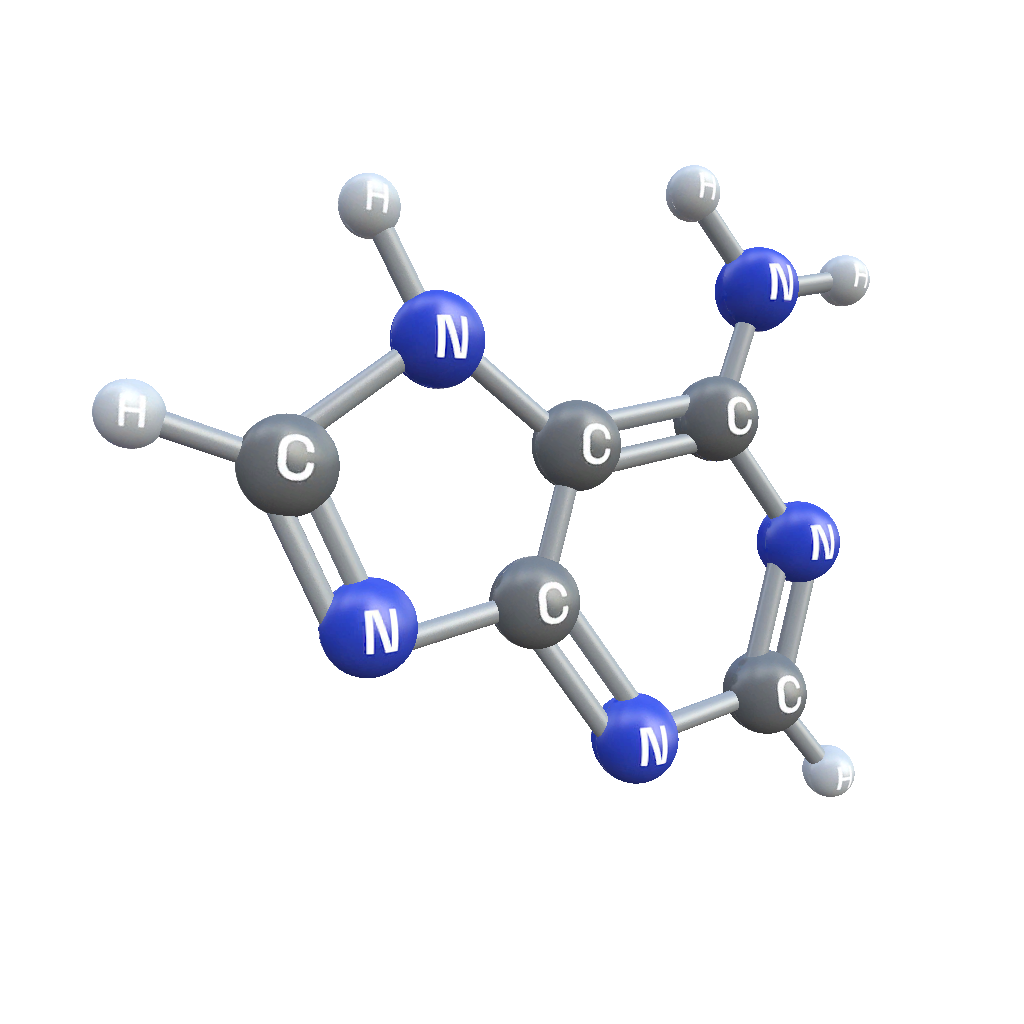The image is an educational diagram depicting a molecular structure, suitable for a textbook or manual. The molecule is illustrated with various small spheres labeled with the letters H (Hydrogen), C (Carbon), and N (Nitrogen). These spheres are connected by rods representing chemical bonds. Specifically, the H spheres are colored light gray, the C spheres are a darker gray, and the N spheres are a sapphire blue. The molecule consists of 15 spheres in total, with connections visible at five open-ended points and two main bodies linked at the center. The diagram shows single bonds running from H to N and C to N, with occasional double bonds appearing between some of the C and N spheres. This detailed visualization helps in understanding the intricate connections and structure of the compound.